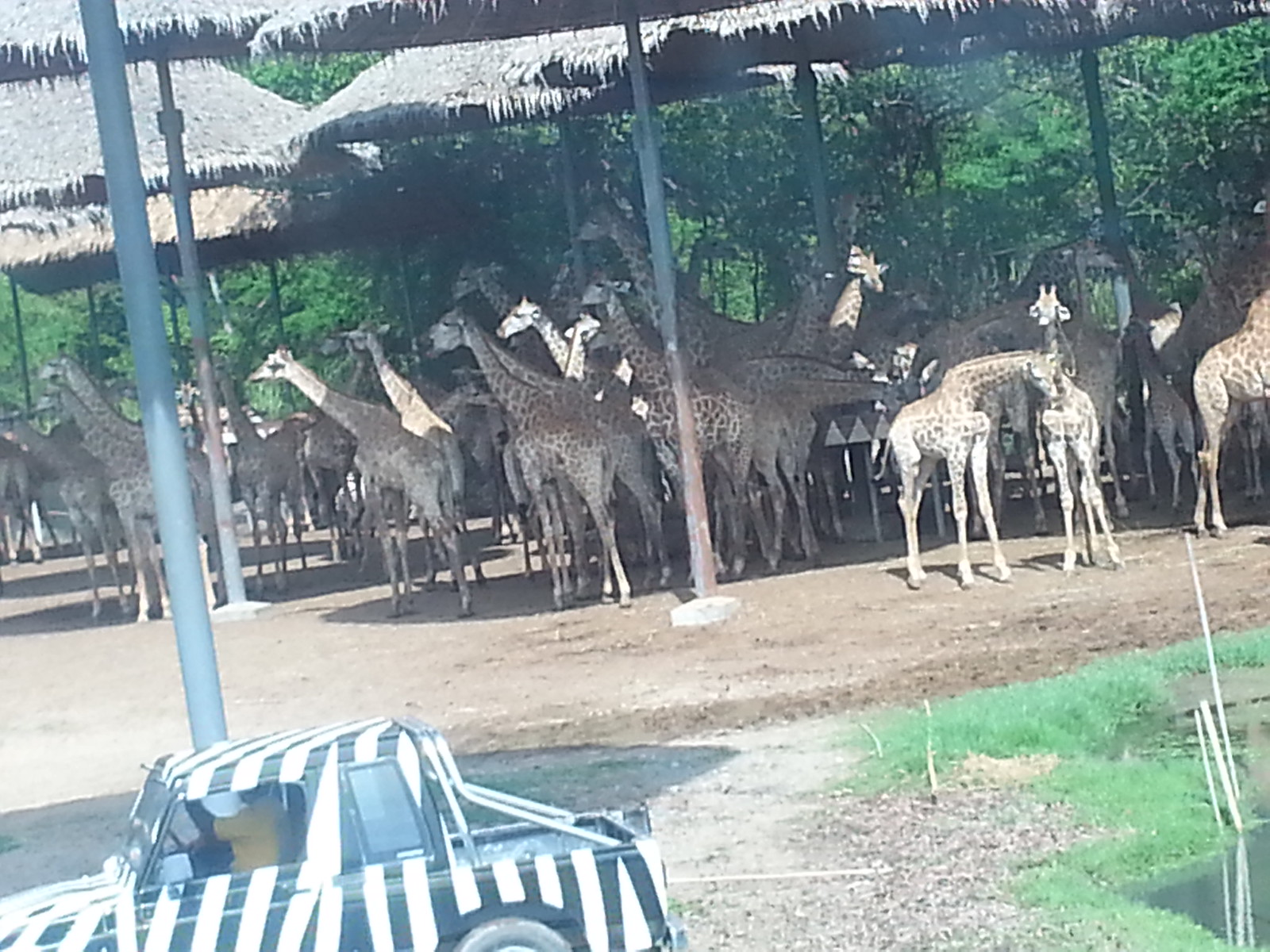The image depicts a safari habitat bustling with juvenile giraffes, standing at about six to eight feet tall, gathered under a series of straw-thatched canopies held up by vertical metal beams. The ground is a dusty expanse, with some areas featuring sparse greenery and pebbles. To the left foreground, a zebra-striped jeep with an open truck bed is being driven by a person in a yellow shirt, moving from right to left. In the right foreground, there is a glimpse of a small pond adorned with green shoreline and rocks. The entire scene, set in a forested area, appears to be contained, with giraffes standing mostly under the shade of the thatched roofs, some of them nibbling at the surrounding trees. The photo has a slightly askew, tourist-snapped quality, adding to its candid and immersive nature.